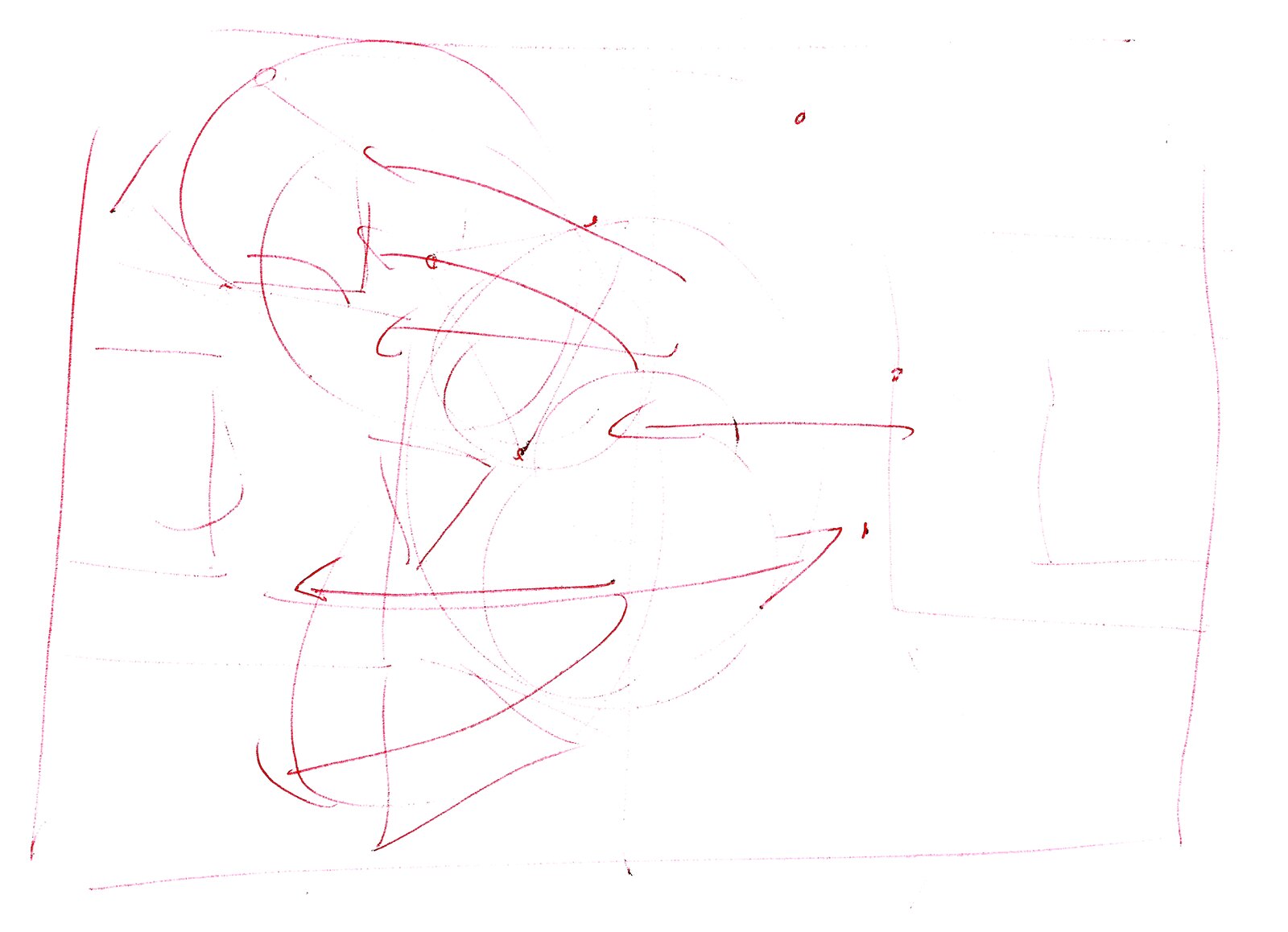This image showcases an intricately detailed drawing, seemingly created with red ink, set against a stark white background. The drawing is framed by a faint red border, with the right-hand edge featuring a slightly squiggled line, adding an artistic touch. 

In the upper left-hand corner of the image, a partially drawn circle is visible, adorned with lines that radiate diagonally inward, creating a sense of depth and motion. Adjacent to this circle is a smaller oval, from which a line extends upwards, suggesting an interaction or connection.

The composition draws the viewer's eye towards the center, which is dominated by an open space lightly shaded in a spherical manner. Arrows surround this central sphere, pointing in multiple directions, hinting at dynamic movement or potential pathways.

Towards the bottom of the image, another sphere is positioned, featuring arrows that extend left and right, and suggesting rotational capability or multi-directional influence. This meticulous arrangement of shapes and lines conveys a sense of organized chaos, inviting viewers to ponder the interconnected elements and their implications.